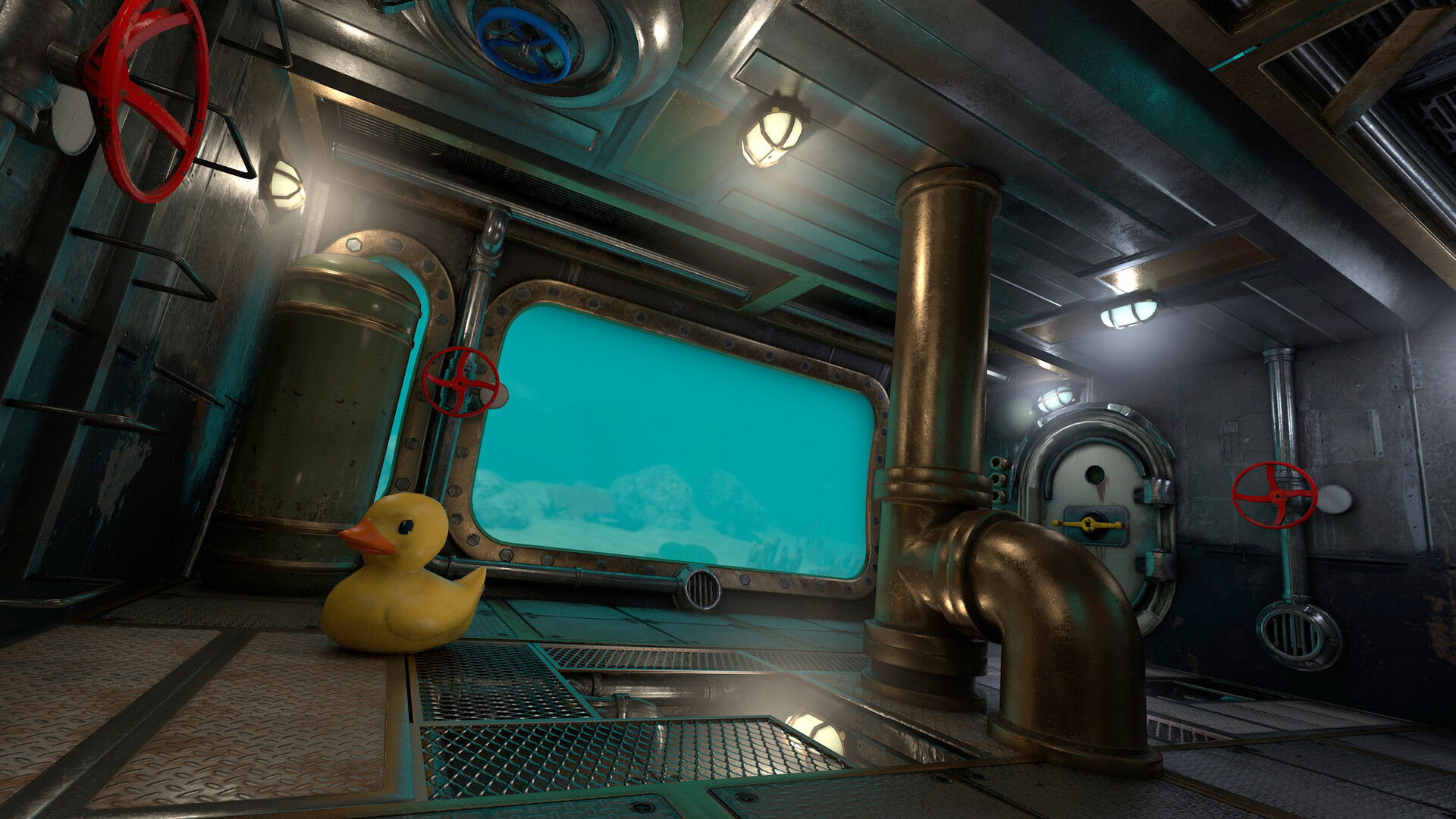The image depicts the inside of what appears to be a submarine or a submersible vehicle, resting on the ocean floor. A large window offers a clear view of the underwater world outside, showcasing rocks, sand, and coral formations. The interior features an array of pipes, including a prominent gold or copper pipe that bends upwards and connects to a vertical pipe leading to the ceiling. Several red, steering wheel-like metal controls are attached to these pipes. On the right side, there is a notably small door that looks challenging for a full-size adult to pass through. Additionally, trap hatch doors with metal handles, and grates forming what looks like a shelf, add to the intricate environment. A whimsical touch is provided by a yellow rubber duck with an orange bill, sitting at the very bottom left of the scene.